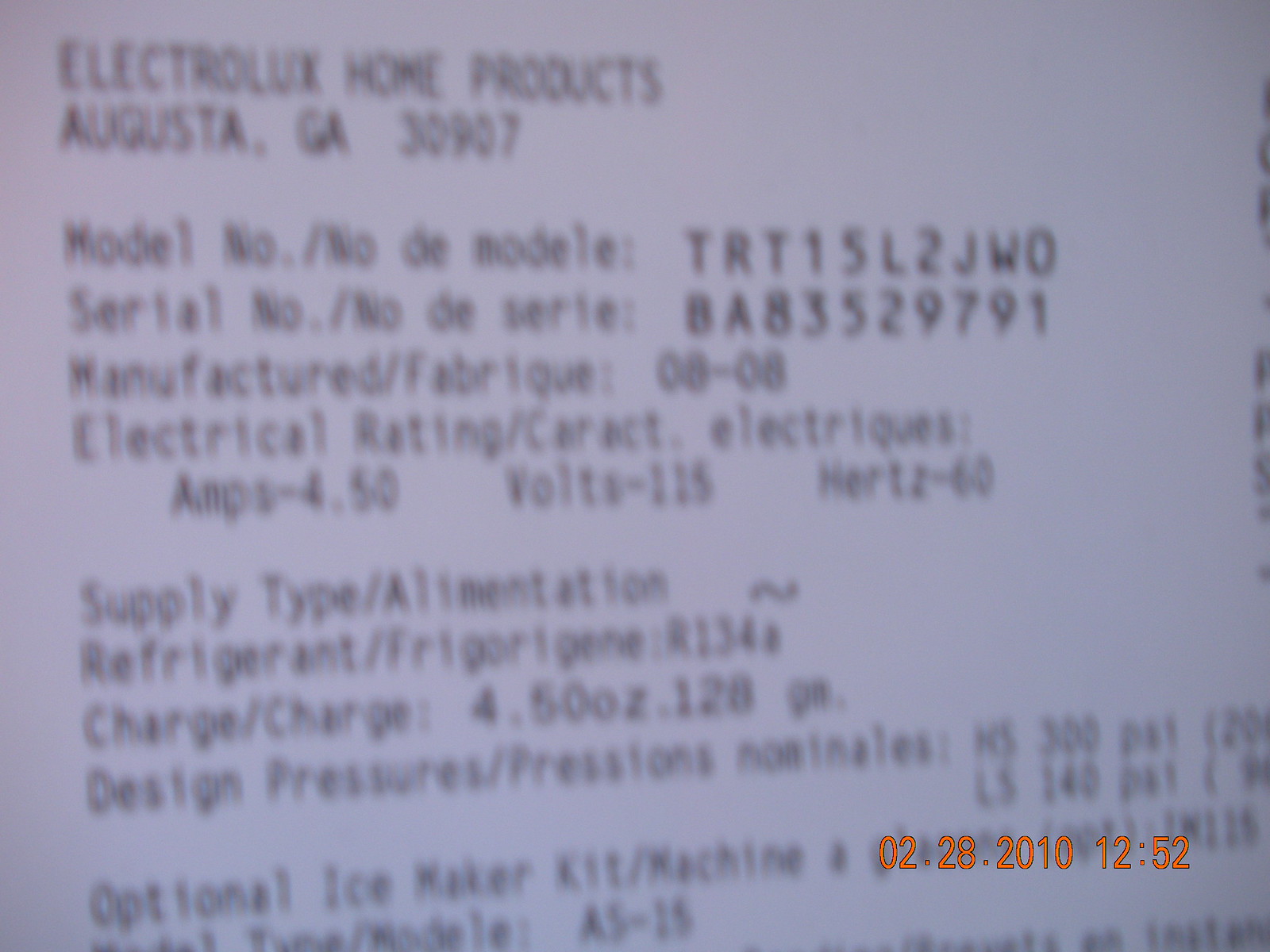The image displays a receipt, albeit out of focus, with a distinct purple hue and black print. At the bottom, there is a date stamp reading "02-28-2010" and a time of "12:52." Despite the blurriness, one can discern the text "Electrolux Home Products, Augusta, Georgia" along with a zip code. Various technical specifications, including serial numbers, model numbers, and manufacturer details, are visible but challenging to decipher due to the lack of clarity. The receipt mentions details about refrigerant type and an ice maker, suggesting it's related to a cooling appliance.